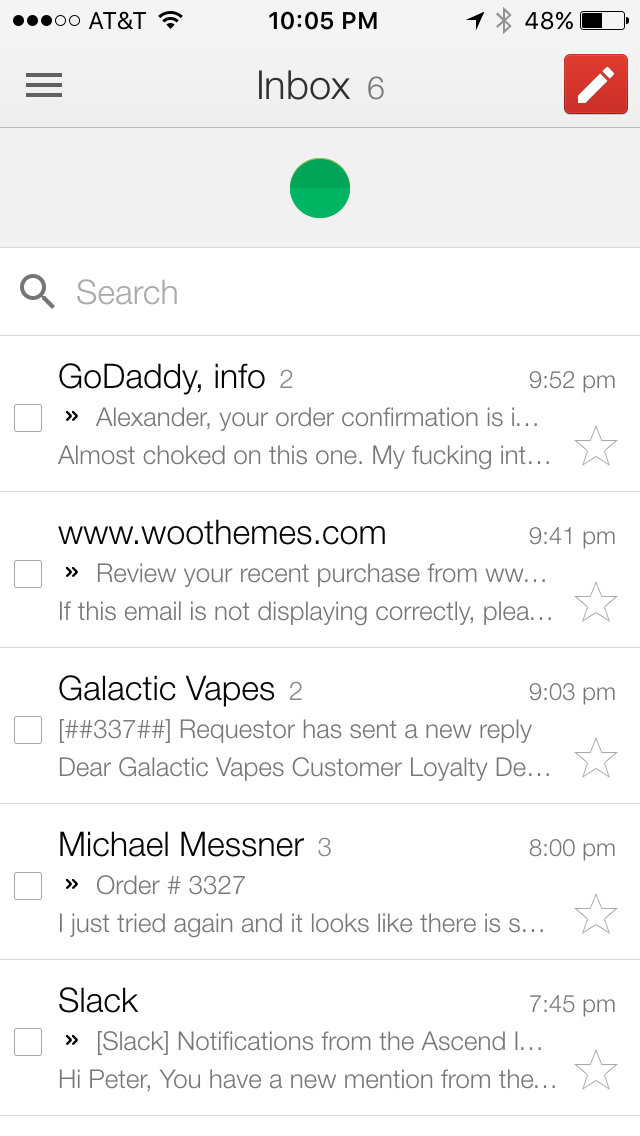This is a detailed screenshot of a Gmail inbox on a phone connected to the AT&T network with Wi-Fi and displaying a 48% battery level at 10:05 p.m. The interface shows 6 new messages indicated by "Inbox (6)" at the top. Underneath that, on the right, there's a red compose button with a pencil icon, followed by a green circle underneath. Next to this circle, there's a search bar with a magnifying glass icon. The list of email senders includes GoDaddyInfo, WooThemes.com, Galactic Vapes, Michael Messner, and Slack. The emails are summarized but not selected, with arrival times around 7:45 p.m. to 9:52 p.m. The entire email interface has a white background typical of a smartphone's email application, affirming the AT&T connection indicated at the top of the screen.